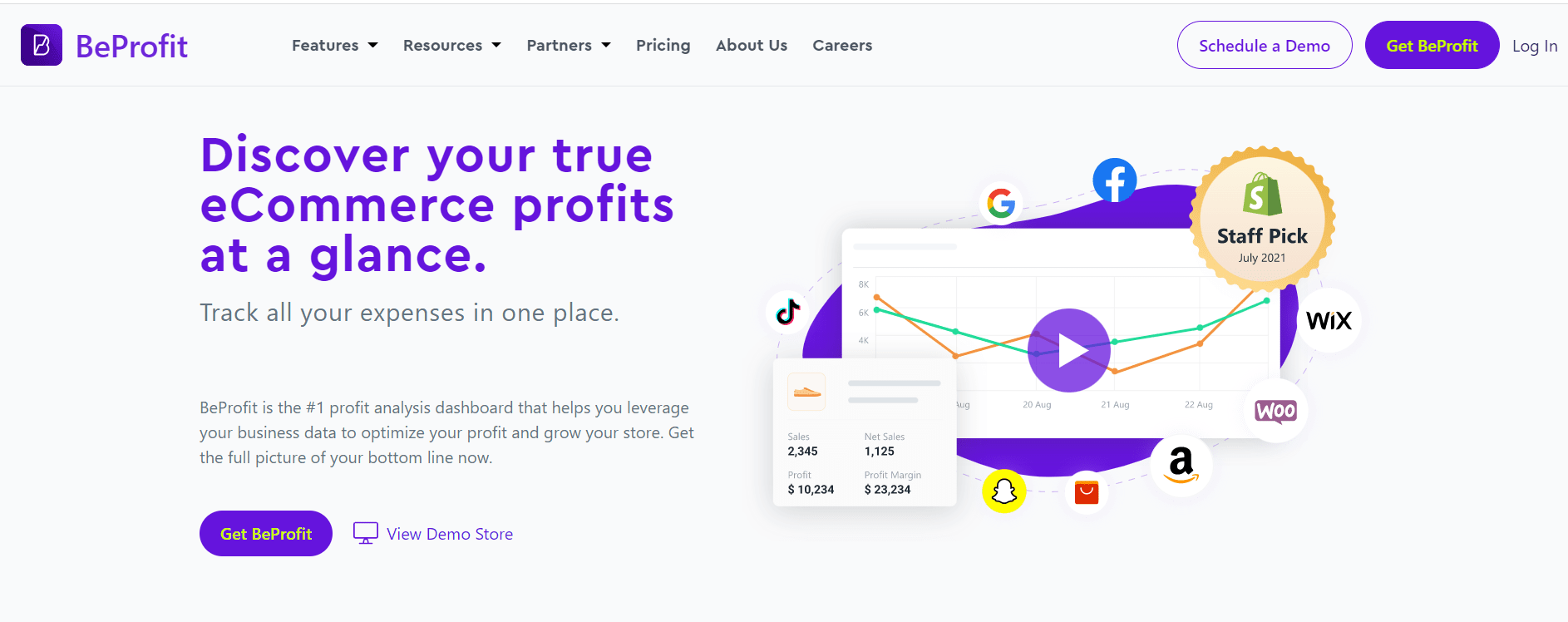The image depicts a web interface with a predominantly light whitish pale lavender background. Dominating the upper portion is a banner bar featuring a user interface for a service named "Bee Prophet," with both words capitalized. On the left side of the banner is a square icon with rounded edges, containing a white bee silhouette. 

Following the icon, the name "Bee Prophet" is displayed prominently. The navigation bar to the right of the name includes several menu items in black font: "Features" with a drop-down menu, "Resources" with a drop-down menu, "Partners" with a drop-down menu, "Pricing," "About Us," and "Careers."

Further to the right, within the banner, is an oval outline in purple with the text "Schedule a Demo" written inside, also in purple. Adjacent to this is a purple button with white font that reads "Get Bee Prophet," and next to it, in purple font, is the word "Login."

The largest text on the image is in purple, reading "Discover Your True Ecommerce Profits at a Glance." To the right of this text block, there appears to be an embedded video player, likely designed to provide additional information to the viewer.